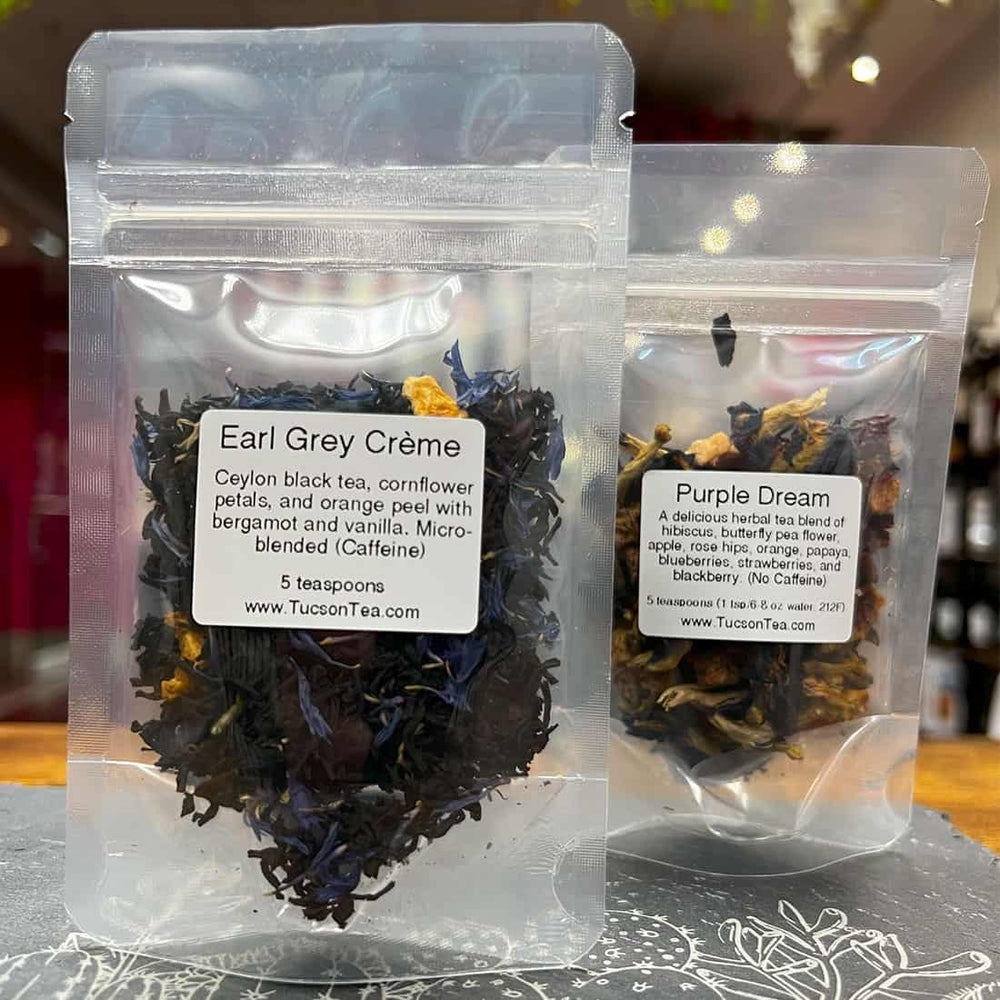This color photograph, in perfect square format, showcases two upright, shrink-wrapped plastic bags of dried tea, positioned one in front of the other on a light gray wood-grain table. The tea bag in the front, leftmost position contains purplish-blue and yellow shavings and features a clear, white label that reads "Earl Grey Cream," detailing its ingredients: Ceylon Black Tea, Cornflower Petals, and Orange Peel with Bergamot and Vanilla. It specifies "Microblended Caffeine" and the quantity "5 teaspoons," along with the URL "www.tucsontea.com." The slightly smaller bag on the right, filled with multicolored shavings predominantly green and yellow, carries a label titled "Purple Dream." This label describes it as an herbal blend of hibiscus, butterfly pea flower, apple, rose hips, orange, papaya, blueberry, strawberries, and blackberry, stating "No caffeine." The label includes mixture instructions and the same URL. Both bags have a tear strip at the top and are placed on a gray and white mat. The background hints at an out-of-focus store interior, emphasizing the clarity and realism of the product in the foreground, in a style best described as photographic representationalism.